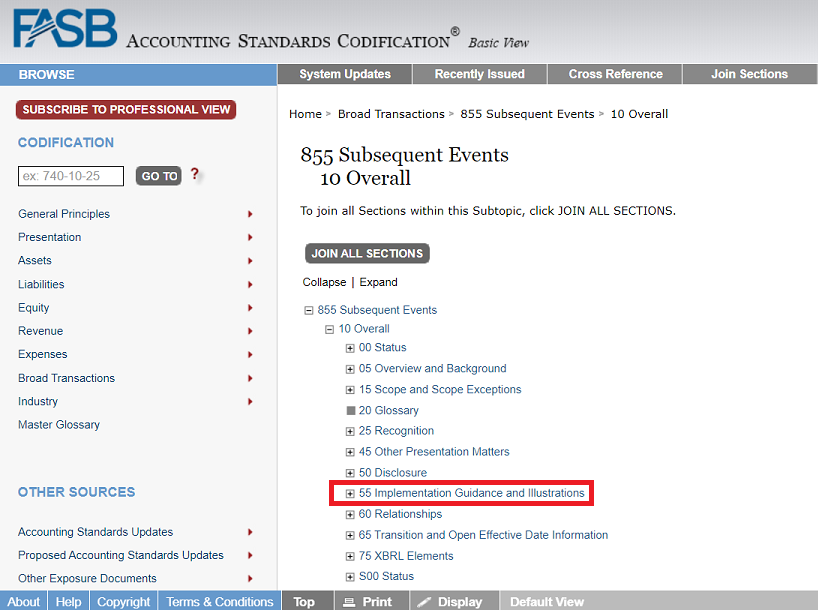The image is a detailed screenshot of the FASB Accounting Standards Codification website. At the very top, there's a gray menu bar that clearly displays the FASB logo and the title "Accounting Standards Codification." 

Below the menu, there is a navigational bar featuring several options: "Browse" which is currently active and highlighted in blue, while the other options like "System Updates," "Recently Issued," "Cross-Reference," and "Joined Sections" are in gray. The "Browse" section has been expanded, showing various suboptions.

On the left side, under the "Browse" button, there is a noticeable blue "Subscribe to Professional View" button followed by the word "Codification" also in blue. Below these, there is a search box and a list of topics including "General Principles," "Presentation," and "Assets," each accompanied by toggle buttons to expand their categories. This list continues with several other accounting-related topics.

Towards the middle-right of the screen, the user has selected a specific section titled "855 Subsequent Events, 10 Overall." Within this section, various bullet points are listed, with one specific item outlined in a red box reading "55 Implementation, Guidance, and Illustrations."

At the bottom of the screenshot, additional menu options in blue include "About," "Help," "Copyright," and "Terms and Conditions." Adjacent to these, a few more navigation buttons in gray are visible.